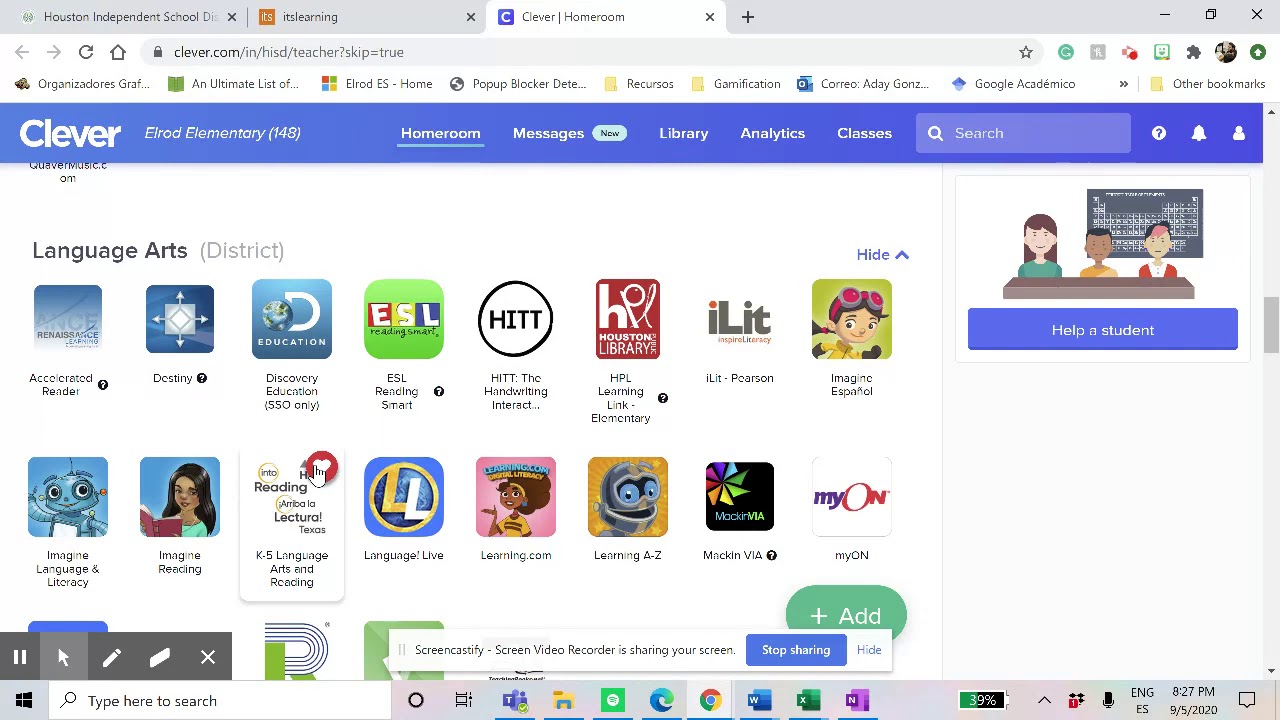A screenshot of a web browser window on a computer displays a light gray header at the top, segmented into multiple tabs. 

1. **First Tab**: 
   - Icon: Present
   - Text: "Houston Independent School" (dark gray, partially faded to the right)
   - Divider: Vertical medium gray line to the right

2. **Second Tab**: 
   - Icon: Present
   - Text: "Itslearning" (dark gray, single word)
   - Close Button: Dark gray "X" on the right

3. **Third Tab** (active/tab in focus): 
   - Background: White with rounded top corners
   - Icon: Present
   - Text: "Clever" followed by a separator and "Homeroom" (both in dark gray)
   - Close Button: Dark gray "X" on the far right

To the right of the tabs, the header contains a series of window control icons: a black "+" sign for opening a new tab, and a cluster of three black icons in the top-right corner representing minimize, maximize, and close actions respectively.

Beneath this header is another lighter gray toolbar. 

- **Left Side**:
  - Navigation Arrows: Medium gray left and right arrows
  - Refresh Button: Dark gray
  - Home Icon: Dark gray

- **URL Bar**:
  - Left Side: Dark gray lock icon
  - Text: "Clever.com/IN/HISD/teacher?skip=true" (black text with the path in medium gray)
  - Right Side: Black star icon for bookmarking

To the right side of the URL bar, there is a variety of colorful icons representing different browser extensions or tools.

Below this area, the browser displays a bookmarks bar. Each bookmark shows an icon on the left followed by its corresponding label in black text.